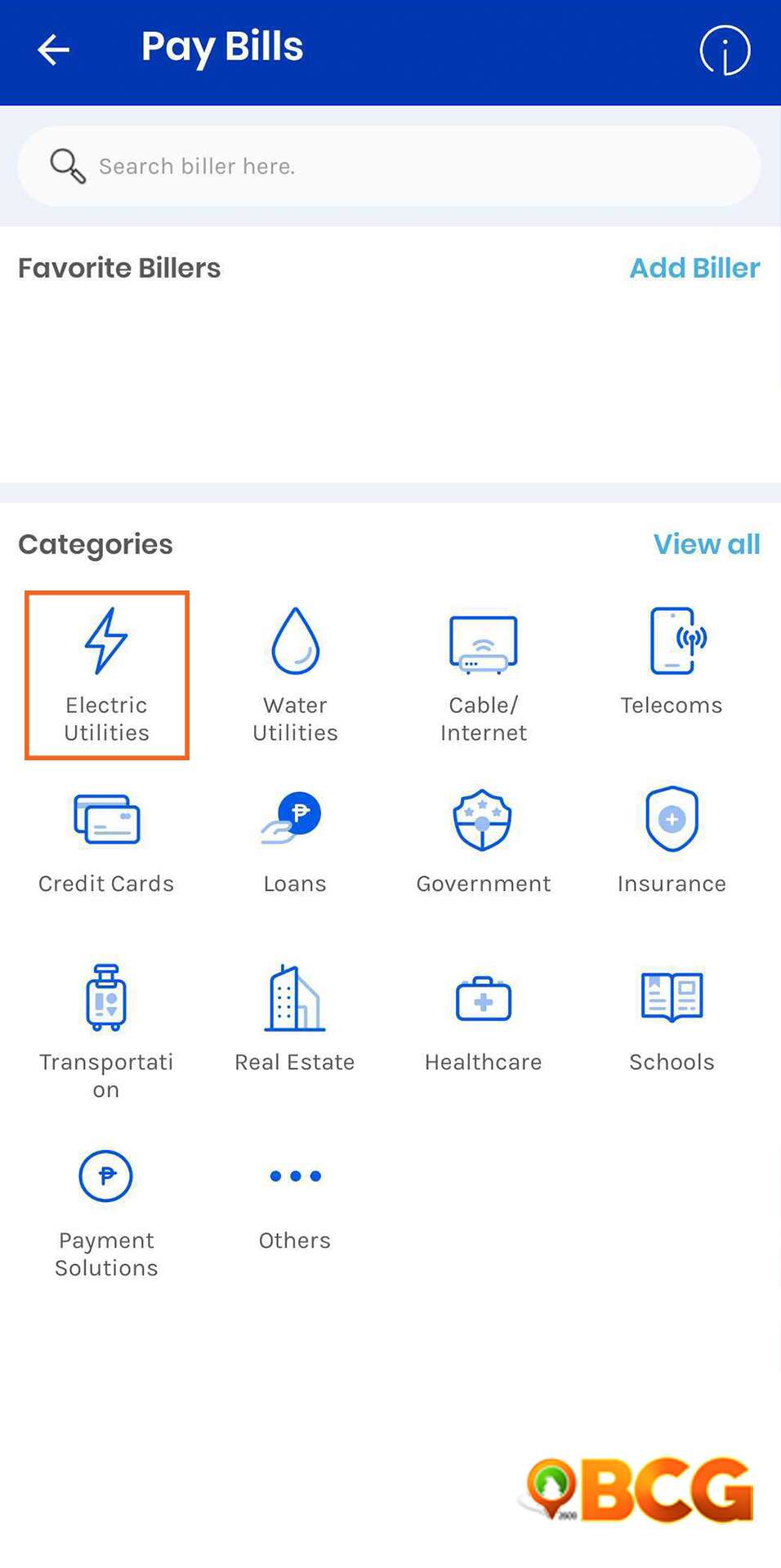This screenshot depicts the "Pay Bills" webpage with a clean and modern interface. The primary background color is white, providing a crisp and clean look. At the top of the page, there's a dark blue navigation bar featuring the text "Pay Bills" in white font. On the left side of this bar, there's a back arrow icon, while on the right side, there's an eye icon within a circle.

Beneath the navigation bar, there's an off-white search field enclosed within a white oval. This field includes a magnifying glass icon to the left and the placeholder text "Search biller here" in grey font.

Below the search field, a large white rectangle contains the text "Favorite Billers" and a blue clickable option "Add Biller." A thin blue line separates this section from the next.

The section below this highlights various biller categories, labeled "Categories," with an option to "View All." The categories displayed include Electric Utilities (which is highlighted with a red square), Water Utilities, Cable and Internet, Telecoms, Credit Cards, Loans, Government, Insurance, Transportation, Real Estate, Healthcare, Schools, Payment Solutions, and Others.

At the bottom of the screenshot, there's a small watermark with the text "BCG."